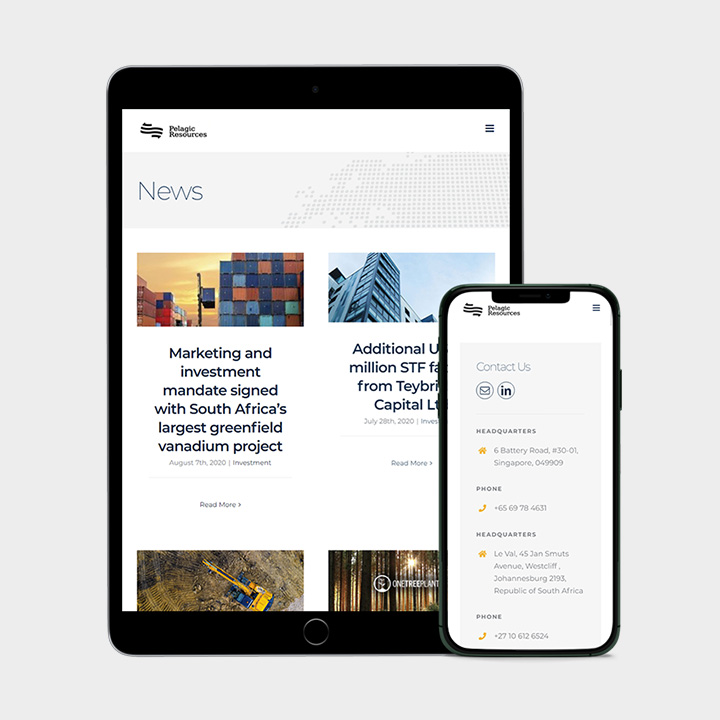The image showcases a digital interface, either an application or a website, for a company named Pelagic Resources. The company's logo, which is stylized to resemble a flag, is prominently displayed. The interface is depicted in two layouts, catering to both tablet and smartphone users.

In the tablet view, a news page is presented featuring four different articles. Two of these articles are fully displayed, while the remaining two are partially visible. One of the fully visible articles is titled "Marketing and Investment Mandate Signed with South Africa's Largest Greenfield Vanadium Project," dated August 7th, 2020, and categorized under Investment. The fourth article is cut off and not fully legible.

The smartphone view presents a "Contact Us" page, displaying the company's headquarters' addresses and contact information. The Singapore headquarters are located at 6 Battery Road, #30-01, Singapore 049909, with a phone number of +65 6978 4631. The South African headquarters are situated at Laval, 45 Jan Smuts Avenue, Westcliff, Johannesburg, 2193, Republic of South Africa, with a contact number of +27 10 612 6524.

Pelagic Resources appears to be an international company with operations in both Singapore and South Africa, specializing in investment and marketing, particularly in large-scale projects such as the greenfield vanadium project mentioned.